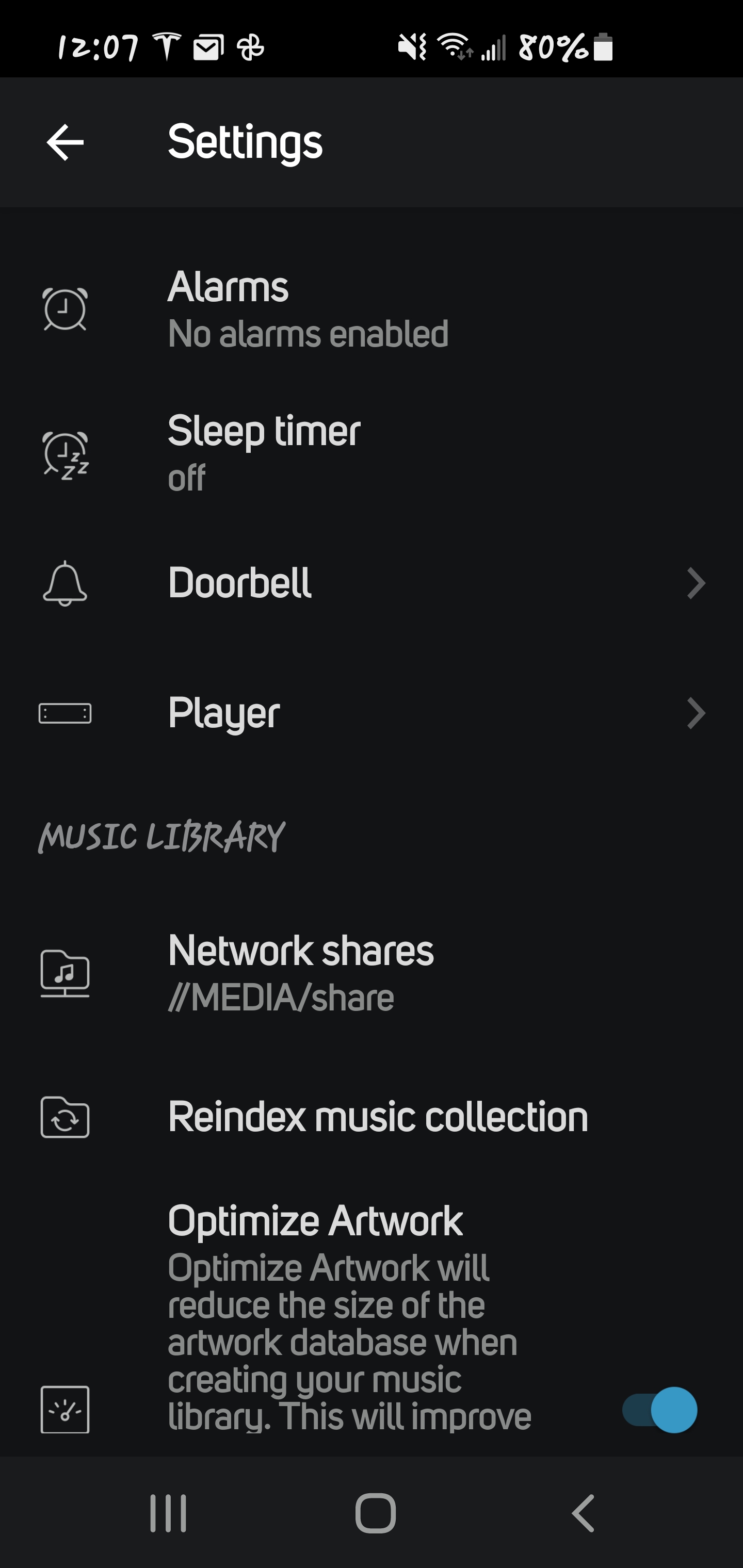The image showcases a cell phone screen with detailed elements and a settings page displayed. The time at the top of the screen reads "12:07". The status indicators show that email notifications are present, sound is turned off, Wi-Fi is connected, cellular signal is active, and the battery is at 80%. The settings page has a black background with white or gray text. There is a back arrow on the top left side of the screen.

The settings menu includes the following items, each accompanied by an icon:
- **Alarms**: An alarm clock icon. The text indicates that no alarms are enabled.
- **Sleep Timer**: An alarm clock with Z's icon. The sleep timer is turned off.
- **Doorbell**: A bell icon.
- **Player**: An icon resembling a bar.
- **Music Library**: An icon that resembles a folder.
- **Network Shares**: A folder icon. The path shown is `//media/share`.
- **Re-Index Music Collection**: This has a folder with a music note icon.

Under the option for "Optimize Artwork," it states: "Optimize Artwork will reduce the size of the artwork database when creating your music library. This will improve..." The sentence is incomplete, but the toggle for this setting is on and highlighted in blue.

Below the settings menu, there are three navigation icons for the phone:
- Three horizontal lines stacked together.
- A square box with rounded corners.
- A backward arrow.

Each setting has its respective icon displayed to its left.